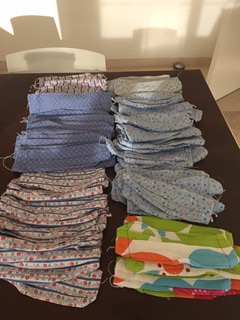This aerial photograph captures a section of a wooden, brown table neatly set with about a hundred homemade cotton face masks, arranged in two vertical rows by their fabric designs. The table is positioned against a cream-colored wall, with light from a nearby window casting soft shadows. Behind the table is the top of a white plastic chair, and to the right, a slightly open tan-colored door is visible. The fabric patterns on the masks are diverse, featuring a mix of blue polka dots, red and green floral prints, and larger geometric prints in green, blue, and orange hues. Each mask displays ear loops, emphasizing their readiness for use. The detailed alignment and variation in prints highlight the handcrafted nature of these protective garments.